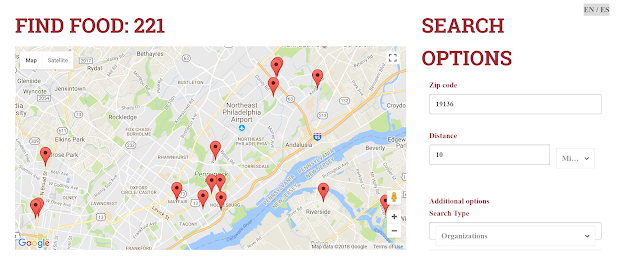This image is a screenshot from Google Maps focused on food search results within a specified area. At the very top, in red text, it reads "Find Food: 221." The primary portion of the image displays a Google Maps interface.

In the top left corner, there are two white boxes with black text, allowing the user to toggle between map view and satellite view. In the top right corner, a white box with a black full-screen symbol enables the user to enlarge the map view. Below this, a cluster of icons includes a gold user symbol and white boxes featuring plus and minus signs, which allow for zooming in and out of the map.

The map itself is dotted with red markers indicating various locations relevant to the user's query. On the right side of the image, "Search Options" and the zip code "19136" are highlighted in red. Beneath this, the search distance is set to 10 miles. Additional options and search type are available in dropdown menus, with "Organizations" selected by the user.

This detailed, descriptive caption provides a comprehensive overview of the Google Maps interface as configured for a specific food search query.